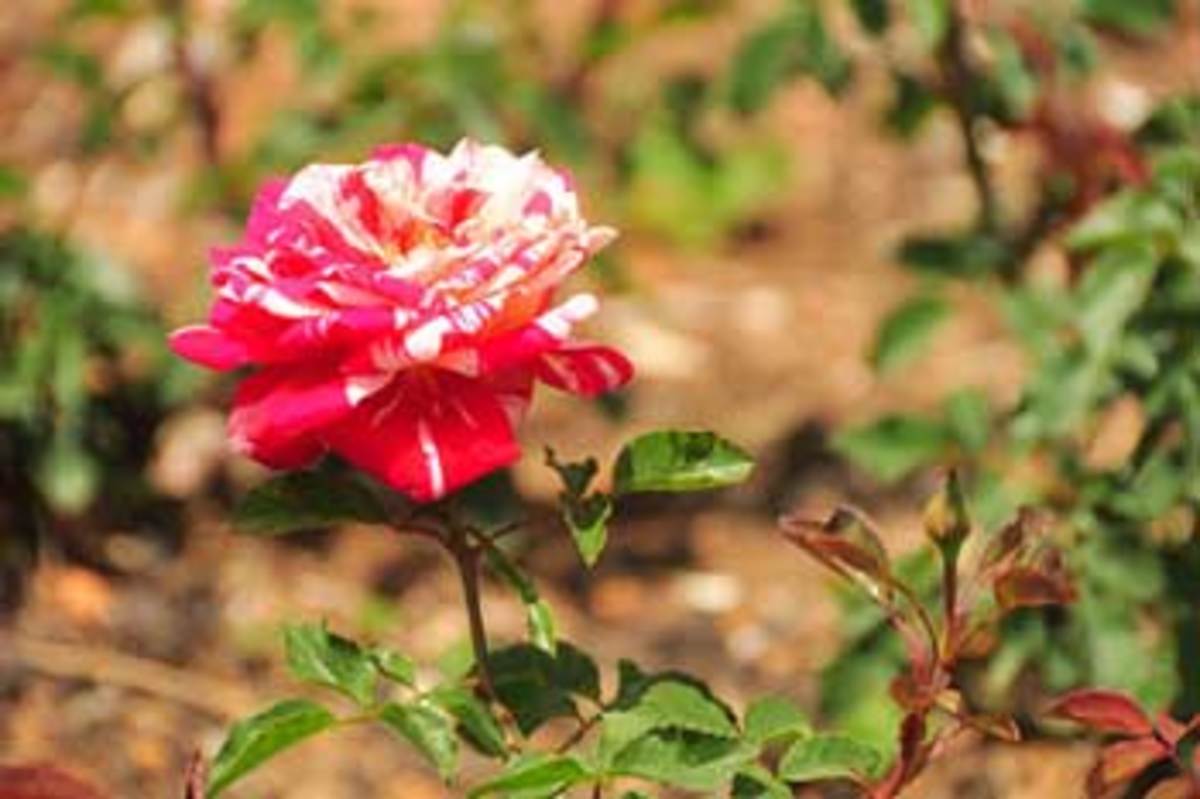This is a color photograph of a vibrant flower, captured in a natural outdoor setting. The central focus is a large red flower, slightly off-center to the left, boasting thin, delicate petals with a mix of red and white streaks, along with blotches of white, shading into pink in some areas. The flower sits on a green stem adorned with plain green leaves. To the bottom right, protruding towards the right side of the image, is a smaller bud on a branch, yet to bloom. The background features a heavily blurred mix of green plants, brown soil, sticks, and some faint white spots, with everything blending into an abstract backdrop that emphasizes the sharp details of the flower and bud in the foreground. The overall color palette includes red, pink, white, green, brown, and touches of black.